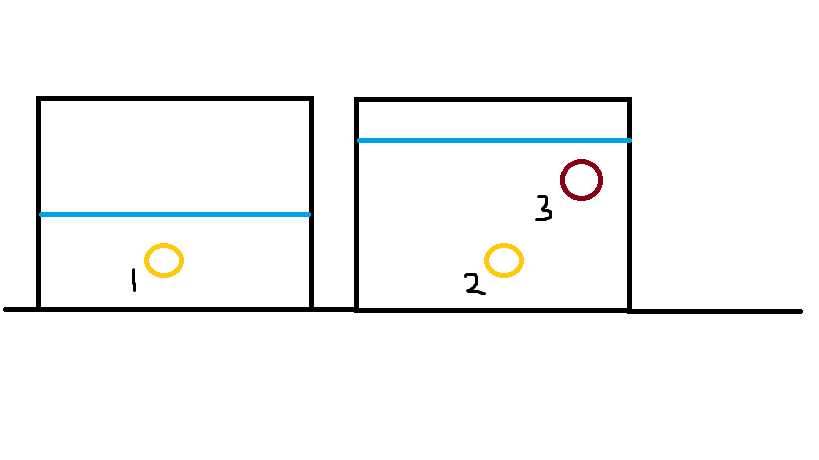Against a stark white background, the image showcases a minimalist illustration composed of a single thin black horizontal line stretching from one edge of the frame to the other. This line serves as the baseline for two squares, which are perfectly aligned atop it. 

The left square features a delicate turquoise blue line positioned slightly below its midpoint. Just above the baseline of this square is a hand-drawn numeral "1" along with a simple, brightly colored yellow circle.

In contrast, the right square has a similar turquoise blue line, but this time drawn much higher, near the top quarter of the square. Near the upper right corner of this square, a maroon circle is found with the numeral "3" adjacent to it. Additionally, a yellow circle, identical to the one in the left square, appears diagonally below the maroon circle, accompanied by the number "2."

This thoughtfully composed image, devoid of any additional text or overt explanation, relies on its geometric simplicity and selective use of color to engage the viewer.